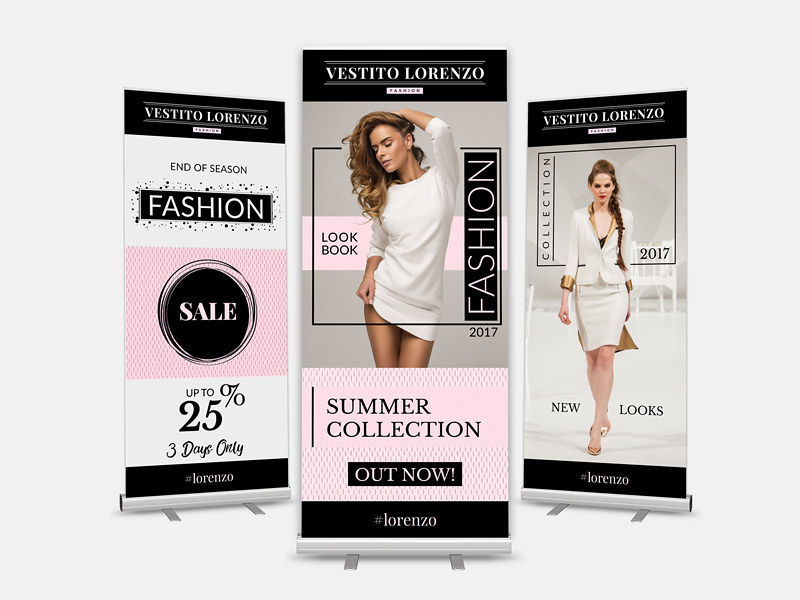The advertisement features three vertical poster stands for Vestito Lorenzo, set against a white background. The central stand showcases a striking image of a woman with long blonde hair draped over her right shoulder. She wears a white dress that reaches her thighs, revealing a bit of her hip on the right side. Above her, "Vestito Lorenzo" is prominently displayed in a black rectangle, followed by the word "Fashion" underneath. The text to her left reads "Lookbook," and below her image, "Summer Collection" is highlighted with "Out Now!" in a smaller black bar. At the bottom, in white lettering, it says "#Lorenzo."

The poster on the right also features a woman, dressed in a white skirt with a black-and-white jacket, posing like a model. It is labeled "Collection 2017" in dark letters, with "New Looks" near her feet.

On the left, the poster is text-centric, announcing an "End of Season Fashion Sale" with discounts "up to 25%" for "three days only." A pink box contains a black circle with the word "Sale," and the bottom also bears the hashtag "#Lorenzo." The stands are supported by flat metal legs, visible at the base of each banner.